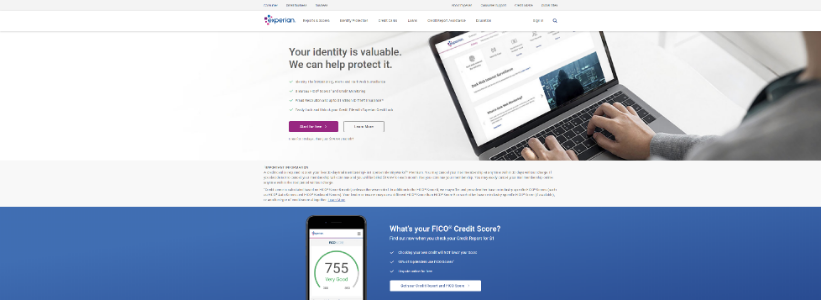The image is a promotional visual for a financial services website, specifically highlighting Experian. The layout is landscape-oriented, mimicking a computer screen composition. At the top, a gray navigation bar is followed by a clean white menu bar showcasing the Experian logo, instantly conveying the brand's identity.

The central portion of the image features an overhead view of an individual typing on a keyboard, with the implication that they are browsing the Experian website. To the left, bold text reads, "Your identity is valuable. We can help protect it," emphasizing Experian's commitment to identity protection. Beneath this message, there is a block of descriptive text further elaborating on their services.

At the bottom of the image, a prominent navy blue bar stretches across, drawing attention with a contrast in color. Positioned slightly left of center is a black cell phone displaying a credit score of 755, a visual testament to a strong credit rating. Adjacent to the phone, the phrase "What's your FICO credit score?" is displayed in crisp white font. Additional copy and a call-to-action button are also present, urging users to engage with Experian's credit monitoring services.

This detailed illustration aims to inform visitors that Experian, a recognized credit reporting agency, offers valuable services such as credit reports, error dispute assistance, and identity protection.